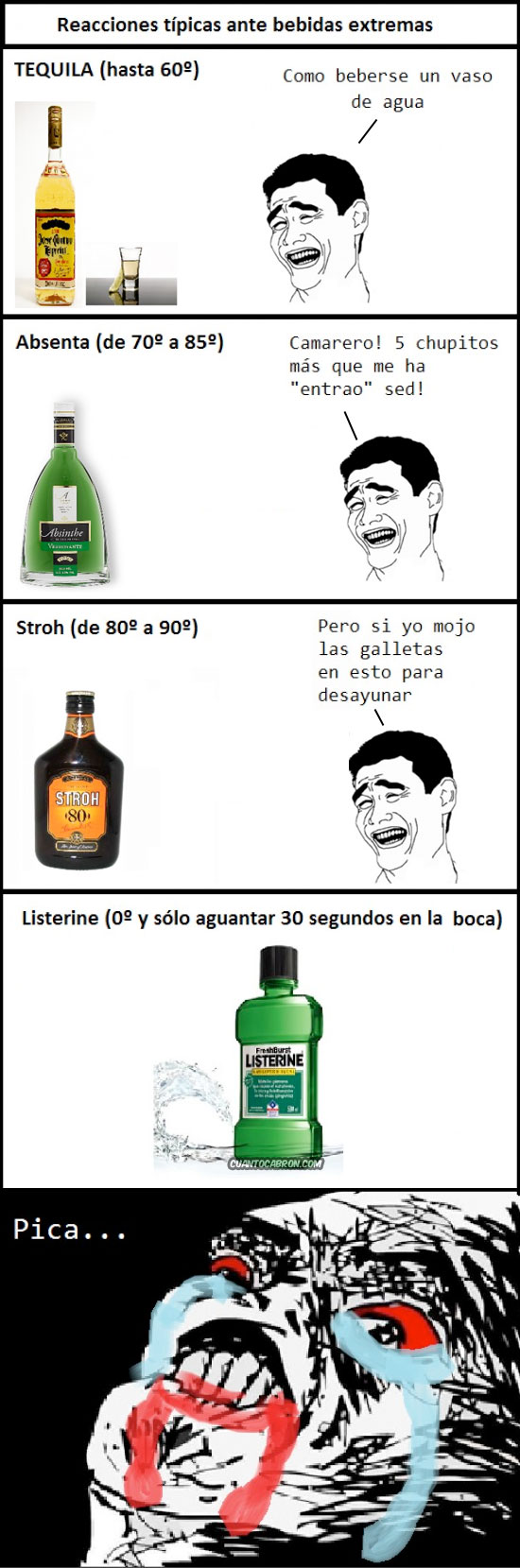The image is a vertically arranged comic strip consisting of six panels. The very thin top panel features black text in Spanish, which serves as the comic's title, possibly referring to different reactions. The first substantial panel below depicts a bottle of tequila accompanied by a shot glass with some tequila in it, alongside a cartoon drawing of a man's face with a speech bubble in Spanish, his expression ambiguous between laughter and crying. The second panel shows a bottle of absinthe with the same cartoon face and another Spanish text bubble. The third panel continues the sequence with a bottle of a darker liquor called Stro and the recurrent cartoon man with more Spanish text. In the fourth panel, there's a bottle of green Listerine; the cartoon man is absent, but Spanish text is present. The final and bottommost panel features a distressed cartoon face, scribbled in black with red coming from the mouth, red eyelids, and blue tears streaming down, contrasting sharply in the predominantly black and white scheme. The overall comic uses a range of colors including black, white, gold, brown, yellow, red, orange, green, and light blue to create a satirical narrative on the effects of different liquids, possibly meant as a meme.